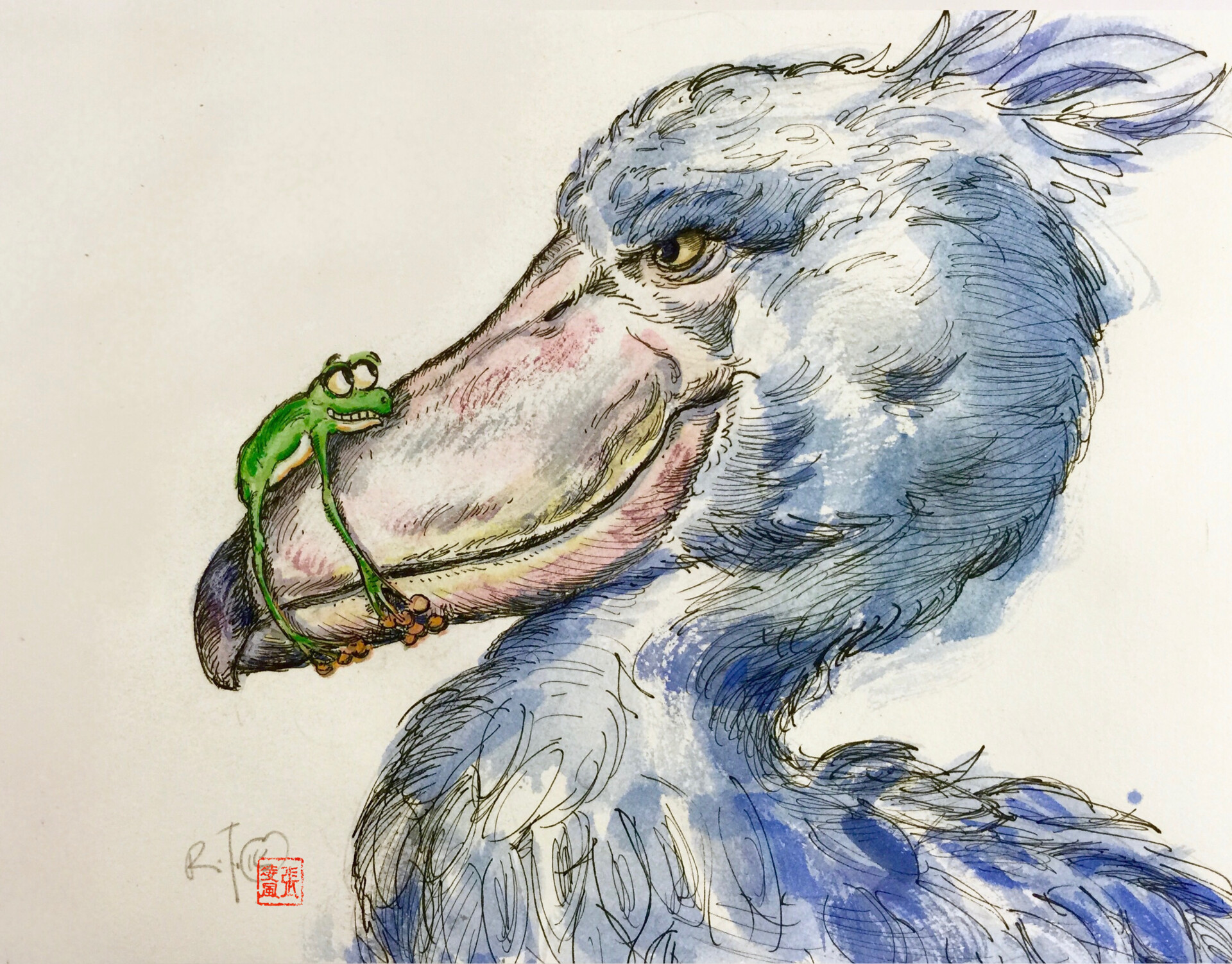This detailed image features an intricately sketched scene of a blue bird and a frog, likely created by a Japanese artist judging by the red square stamp with Japanese kanji and the initials "RT" in the bottom left corner. The bird, depicted in vibrant shades of light and dark blue, has a beak that blends hues of pink and white, and is further detailed with black strokes that illustrate its feathers. Resting atop the bird's beak is a bright green frog with striking orange pads on its limbs and a whitish-orangish underbelly. The frog's large, white eyes gaze upward into the bird's eyes, suggesting a connection or interaction between the two. The background of the artwork is a simple off-white or beige, ensuring that the focus remains on the engaging interplay between the bird and the frog in this evocative piece.